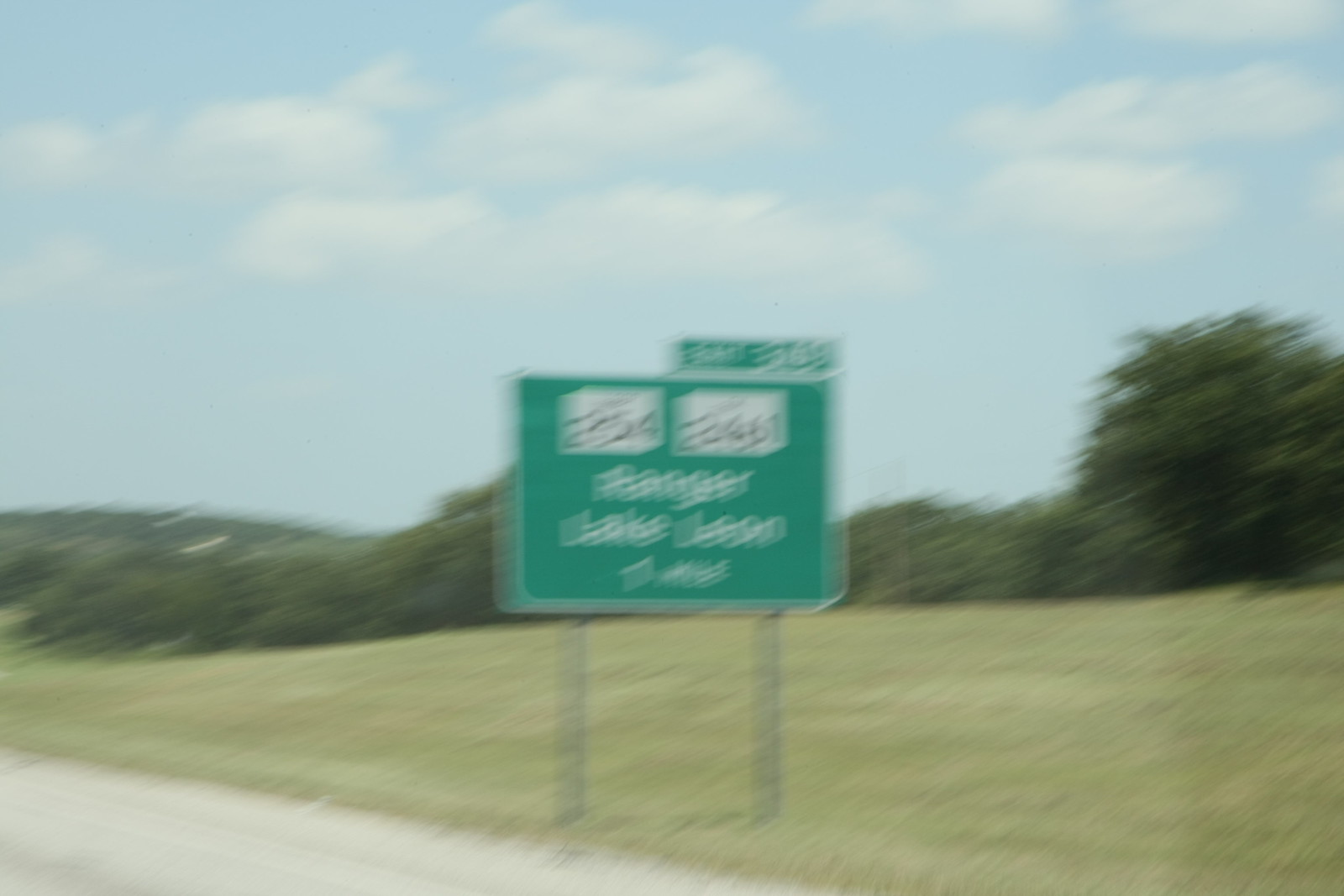In this image, we observe a very blurry outdoor scene likely captured from a moving vehicle, such as a car or bicycle. The perspective suggests the photographer was traveling along a road when the photo was taken. The image partially reveals the road itself, with an adjacent field or open grassy area to the right. This grassy expanse is bordered by what appear to be trees or shrubs, although the blurriness makes it hard to distinguish specific details. Overhead, a light blue sky with patches of clouds is faintly visible. Additionally, close to the road's edge, there is a green road sign; however, due to the blur, the text on the sign is unreadable.